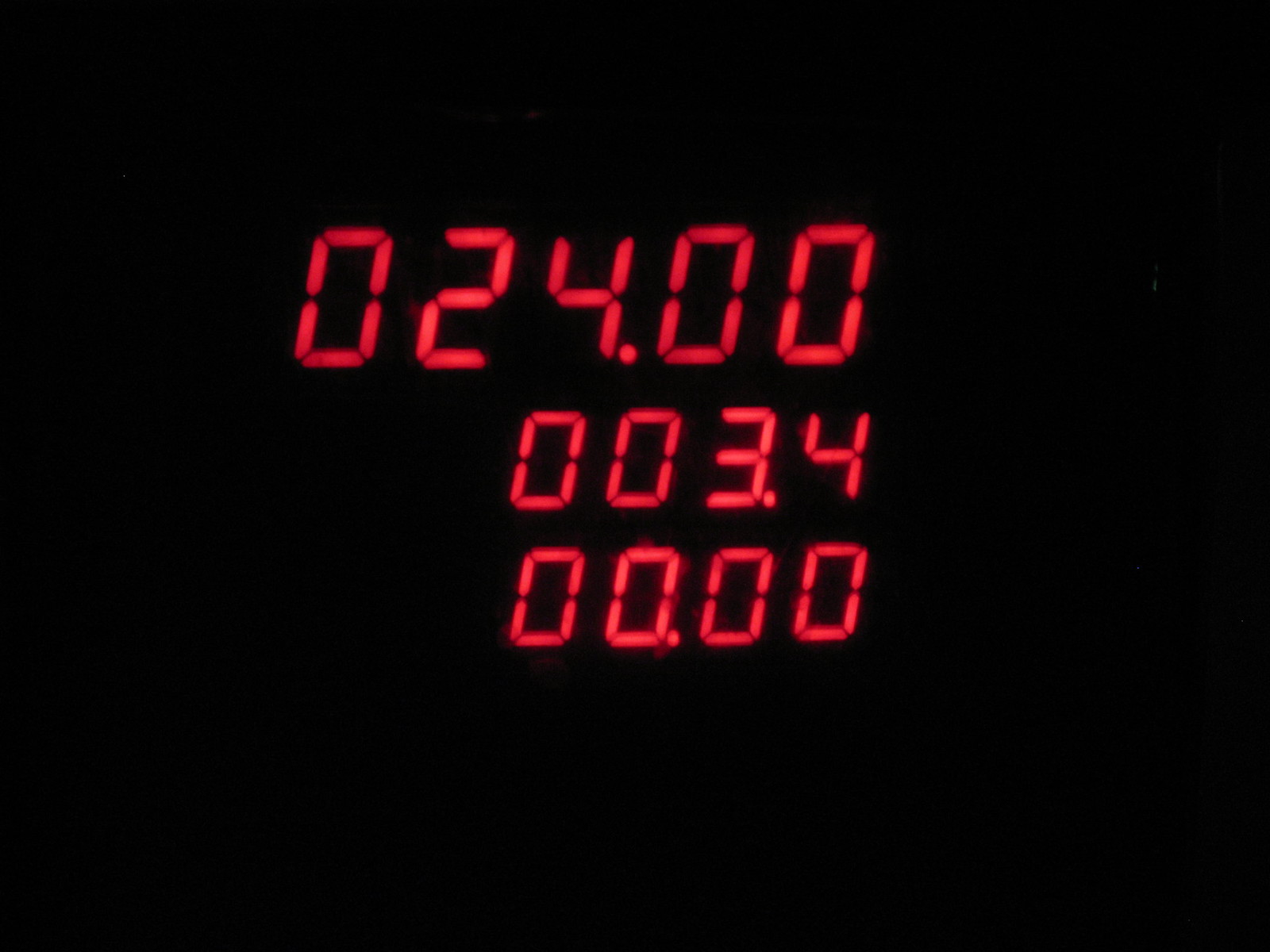In this horizontally-oriented rectangular image, the entire background is a deep, unbroken black, creating a stark contrast that emphasizes the central elements. Prominently displayed near the top center of the image are three vivid red digital numbers, '024.00', glowing brightly against the darkness. Just below these numbers, perfectly centered, the digits '003.4' are illuminated with the same intensity. Directly beneath these figures, another set of numbers, '00.00', is aligned precisely, continuing the pattern of luminous red digital readouts that punctuate the otherwise entirely black scene.